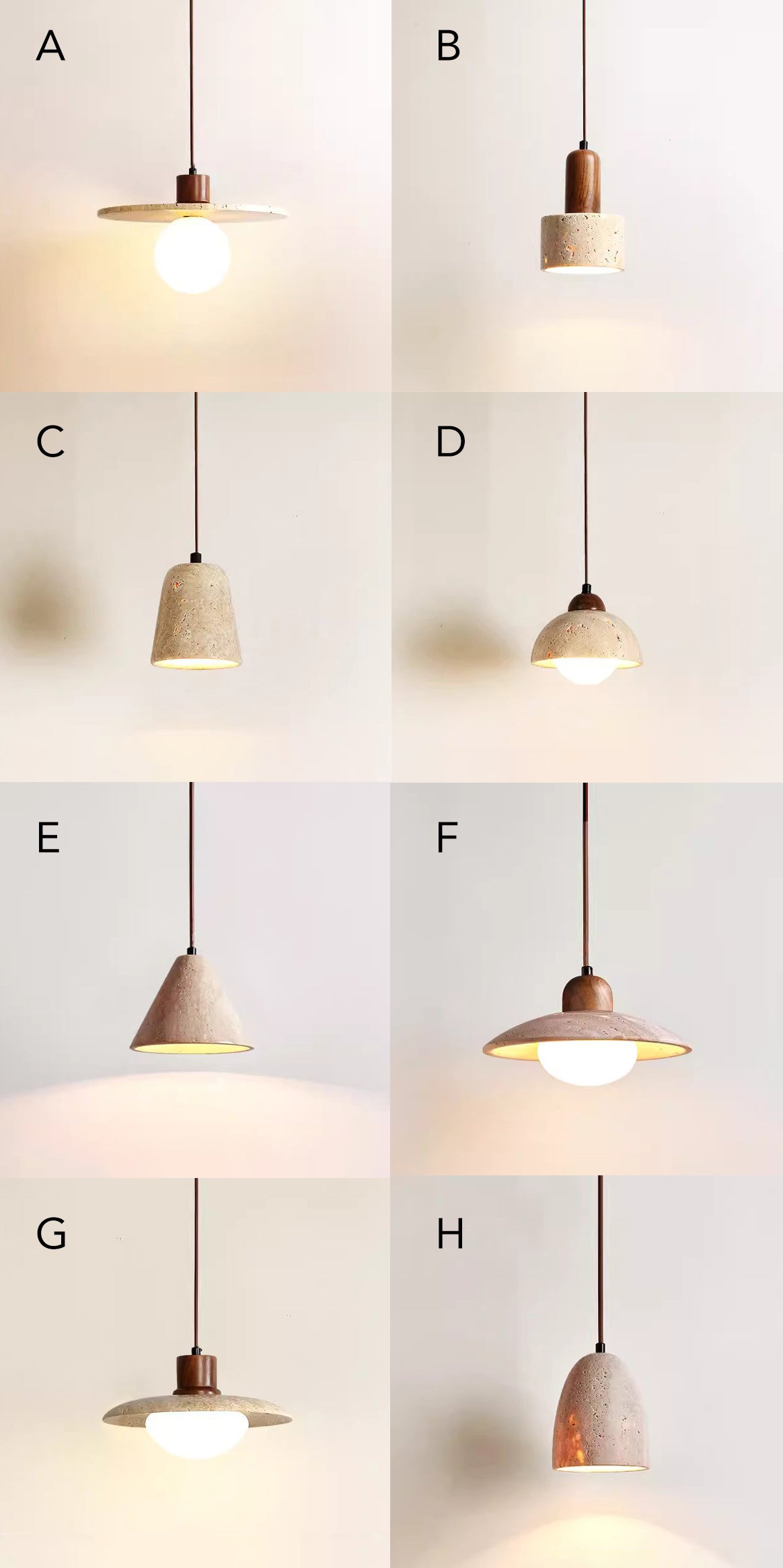The image features eight distinct ceiling pendant light fixtures arranged vertically against a beige background, each with unique designs and shades. Fixture A has an exposed round bulb with a disc-like shade, resembling a saucer. Fixture B features a cylindrical lampshade that fully encases the bulb, noted for its beige tone. Fixture C displays a bell-shaped or thimble-like shade that widens where it exposes the bulb. Fixture D utilizes a semi-hemispherical or half-spherical shade that mostly covers the bulb. Fixture E presents a fully covering triangular or cone-shaped shade. Fixture F is characterized by a large UFO-like saucer shade, with the bulb exposed. Fixture G also has a saucer-shaped shade, but it is smaller than F and has a curved edge. Lastly, fixture H boasts a bell or bullet nose-shaped shade that covers the bulb. All shades vary in design but maintain a consistent color theme, contributing to a cohesive yet diverse display of pendant lighting.